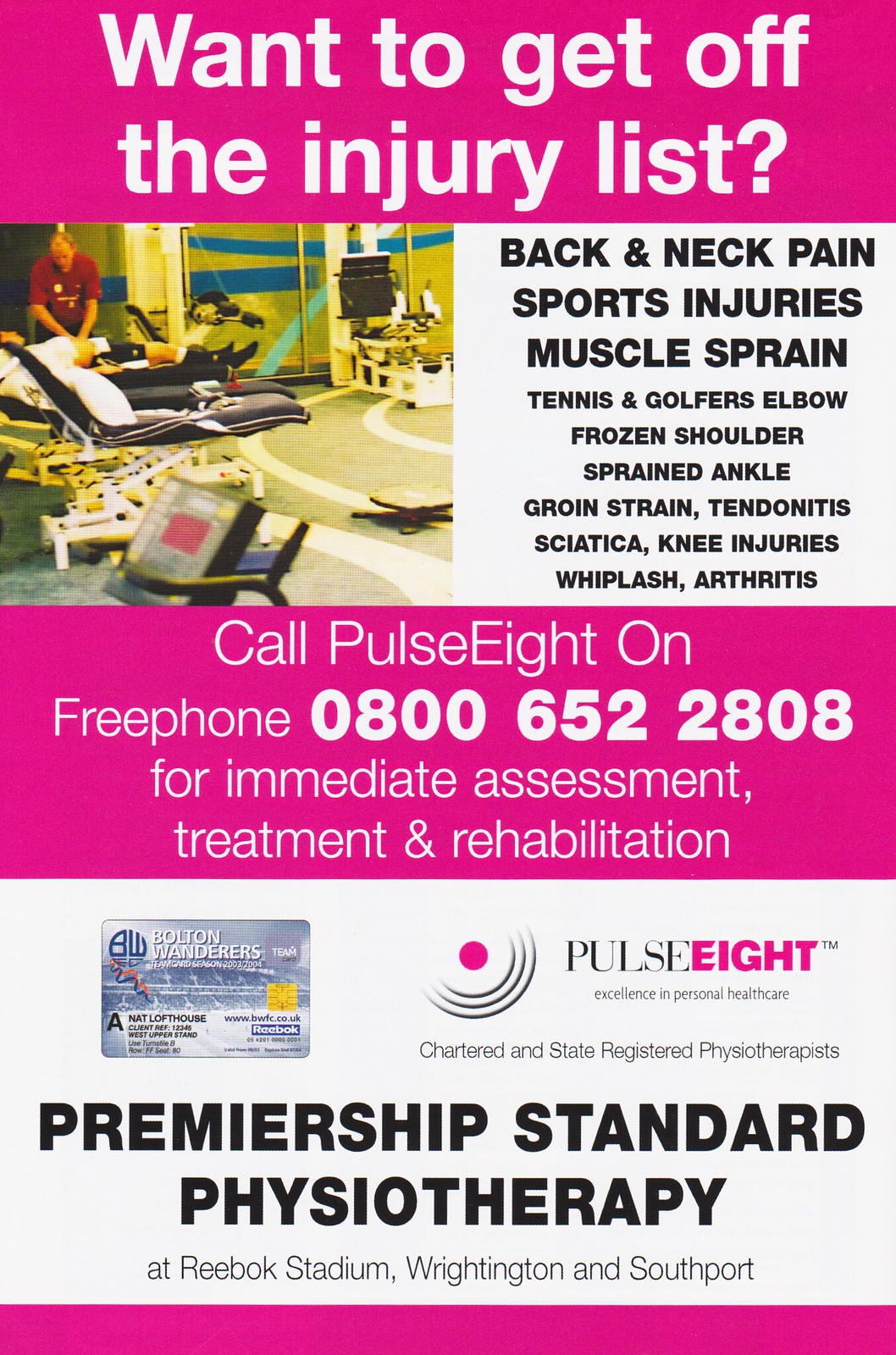The image is a flyer advertisement with a predominantly white background, featuring vibrant pink and white accents. The top section displays a prominent pink banner with large white text that reads, "Want to get off the injury list." Below, the flyer is divided into two main sections. 

On the left side, there's a photograph depicting sports therapy in a room that resembles a gym, with mirrors on the walls, black chairs, and various equipment. The scene captures a person in a red shirt performing a treatment on someone lying on a table. 

The right side lists common conditions treated, beginning with larger black text stating "Back and neck pain, sports injuries, muscle sprain," followed by smaller black text mentioning "tennis and golfer's elbow, frozen shoulder, sprained ankle, groin strain, tendonitis, sciatica, knee injuries, whiplash, and arthritis." 

Beneath this, another pink banner urges readers to call Pulse 8 on free phone 0800 652 2808 for immediate assessment, treatment, and rehabilitation. 

At the bottom of the flyer, there are additional advertisements for Pulse 8 and Bolton Wanderers, highlighting "Premiership Standard Physiotherapy at Reebok Stadium, Rightington and Southport."